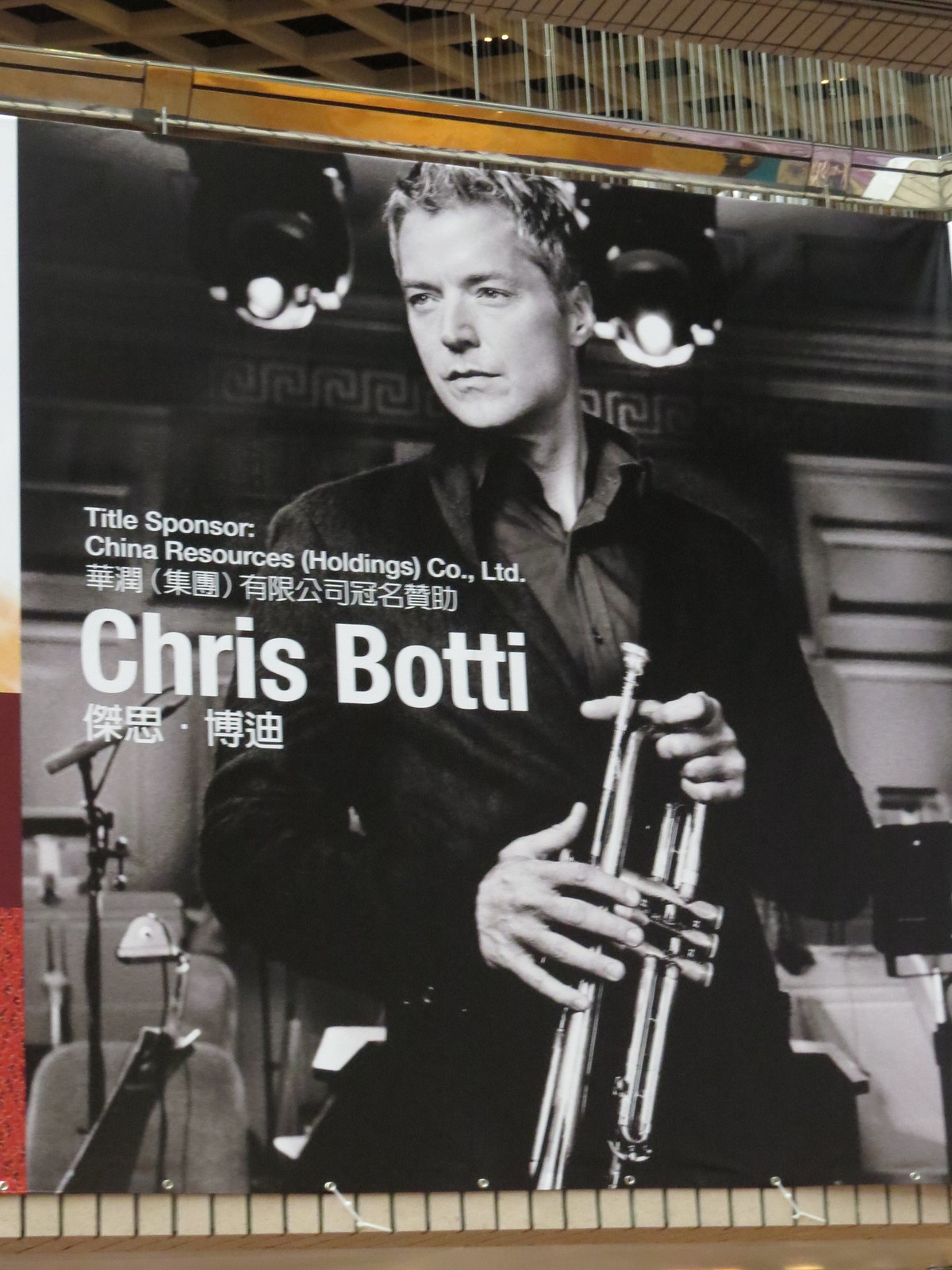The image features a large, black and white poster prominently displayed against a rail, possibly on a balcony or indoors, most likely in a music museum. Central to the image is a white man with blonde hair, dressed in a dark button-down shirt, a suit jacket, and dark pants. He stands stoically, holding a trumpet at stomach height and gazing to the left. Above the poster is a banner, and the text on the poster reads: "Title Sponsor, China Resources Holdings Company LTD," followed by Chinese characters. Below this, in large white text, is the name "Chris Botti," again accompanied by Chinese characters. The setting appears to include elements suggesting a stage, such as a microphone and some chairs on the left, while hinting at interior furnishings on the right. The color scheme of the scene includes black, white, various shades of gray, red, maroon, tan, and brown. This well-arranged presentation emphasizes the musician, Chris Botti, as the focal point of the display.